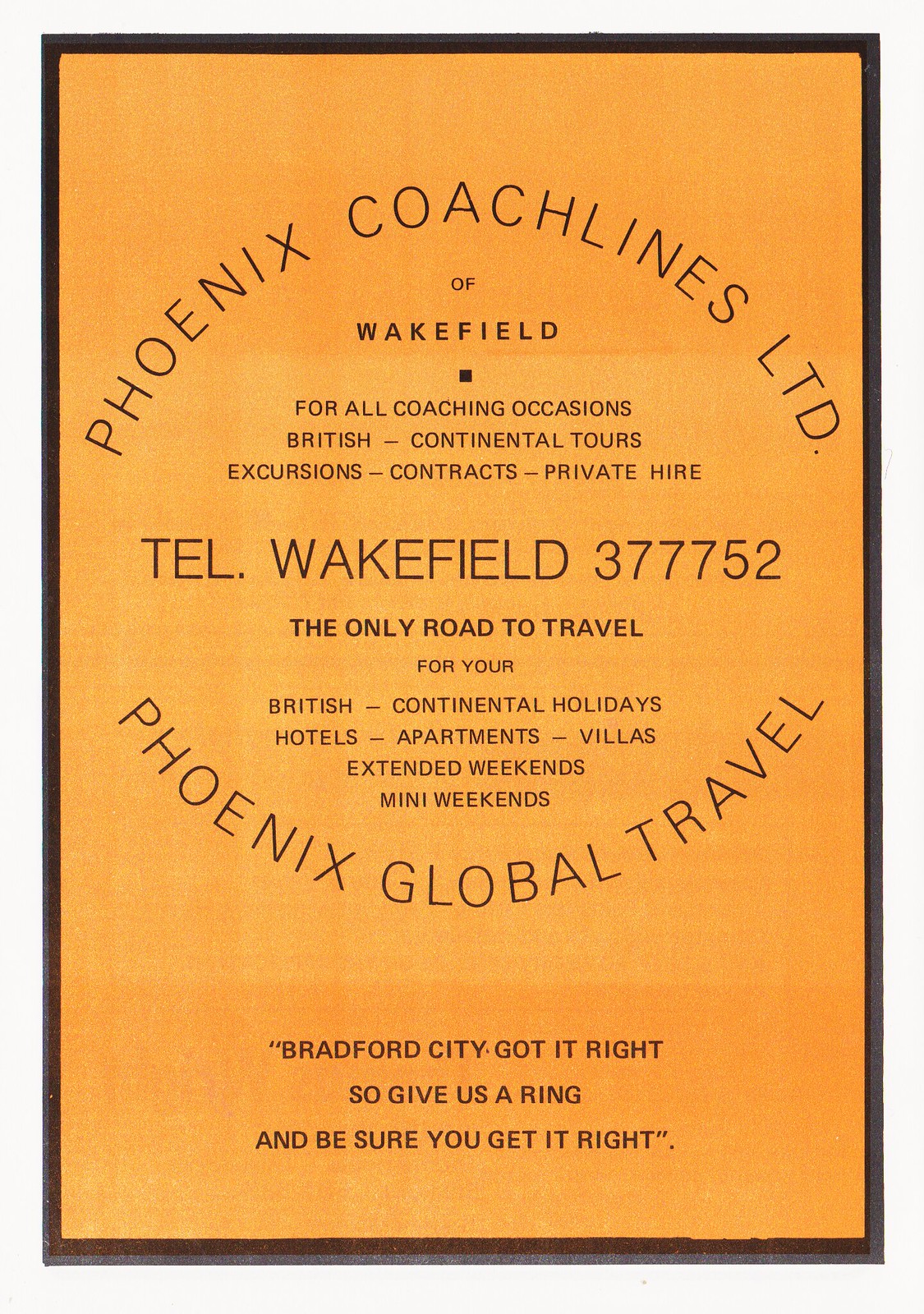This image is a rectangular advertisement with a black border and an orange-yellow background. It prominently features black text in a circular formation at the top and bottom. The top half reads "Phoenix Coach Lines Limited" in an arched layout, while the bottom half circles back with "Phoenix Global Travel," enclosing the inner message.

In the center, the text highlights the services offered: "of Wakefield for all coaching occasions, British continental tours, excursions, contracts, private hire. Telephone Wakefield at 377752." It further emphasizes, "The only road to travel for your British continental holidays, hotels, apartments, villas, extended weekends, mini weekends."

At the bottom of the advertisement, in prominent black text, it states, "Bradford City got it right, so give us a ring and be sure you get it right."

The overall message is clear and promotional, devoid of any images, focusing solely on the detailed, text-based advertisement offerings from Phoenix Coach Lines Limited and Phoenix Global Travel.